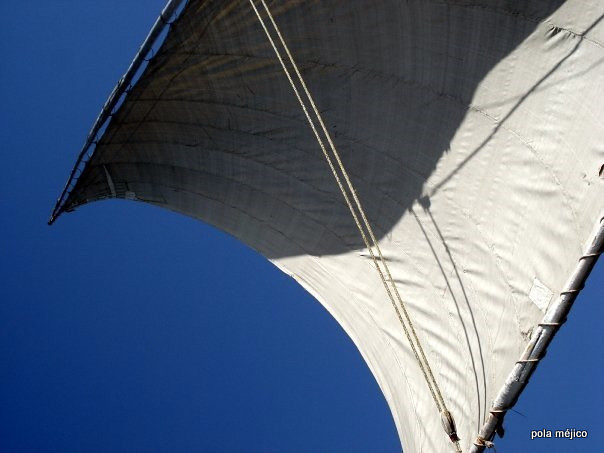The image depicts a square sail of a sailboat, angled slightly to the right, with a pronounced curve extending from the 9 o'clock position down to the 6 o'clock position. The top half of the sail is black, while the bottom half is white, and the sail itself is thick and substantial. A shadow diagonally casts over the upper portion of the sail, extending towards the top right corner, indicating bright natural sunlight against a deep blue sky. The sail is attached to a top rail with rings, and a pulley cord runs from the top center to the bottom right. At the bottom of the sail, it is secured with a rope wrapped around a bottom rod. In the bottom right corner of the image, there are small letters spelling out "P-O-L-A, Pola" and "M-E-J-I-C-O, Mexico." The image is vivid and clear, highlighting the stark contrast between the sail and the blue sky.